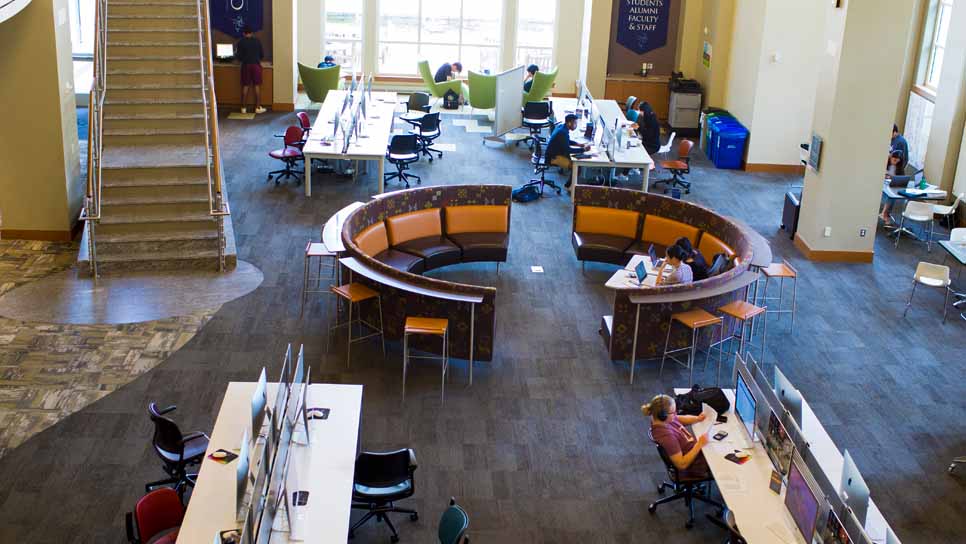This horizontally aligned rectangular image captures an indoor scene likely set in a university library or office during the day, illuminated by a blend of natural and artificial light. The photograph appears to be taken from an elevated perspective, possibly a floor above, overlooking a multi-functional work area. 

On the upper left side, a flight of stairs ascends, adjacent to several open windows that introduce a generous amount of daylight from the upper center to the upper corners of the frame. The floor below is comprised of dark wood tile.

Dominating the lower portion of the image are long wooden desks lined with multiple computer monitors, with a couple of people working at these stations. On the lower right, a woman in a purple t-shirt is focused on her screen, while on the far end of this area, a man sits engaged at one of the desks. 

Near the center of the room is a distinct circular seating arrangement, split into two semicircular sofas with individuals working on laptops perched on small tables. Surrounding this central seating are additional stools paired with desks, enhancing the functional versatility of the space. 

Further to the far end, against the backdrop of a large window, green chairs are occupied by a handful of people engrossed in reading, contributing to the studious atmosphere. The overall scene suggests a well-utilized and efficiently designed space, blending individual workstations with communal areas, typical of a modern university library.